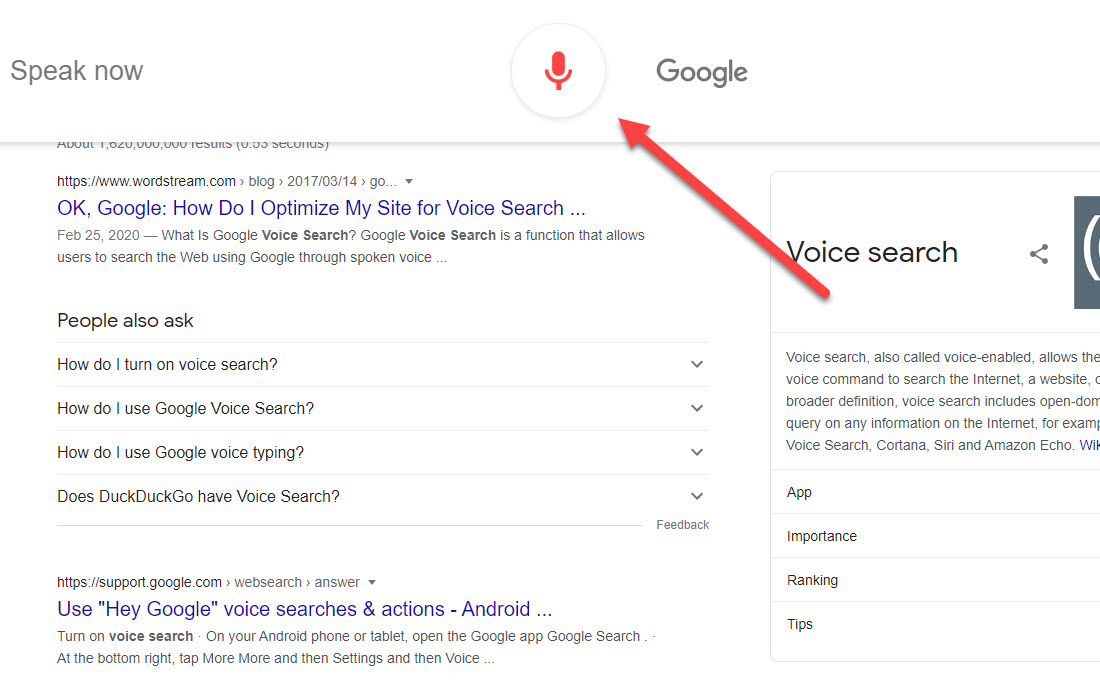The image displays a comprehensive guide to using Google Voice Search, presented in a clean and structured format. The top left corner of the image features the text "Speak now" on a white background. Adjacent to it, on the right, is a white circle with a gray border encasing a red microphone icon, with a red arrow pointing towards it, labeled "Google."

Beneath this, the image transitions into a search result page, showcasing WordStream's website with the query, "Okay Google, how do I optimize my site for voice search?" dated February 29, 2020. Below this result is a brief explanation of what Google Voice Search is: "Google Voice Search is a function that allows users to search the web using Google through spoken voice."

Further down, there is a "People also ask" section with common related queries:
- How do I turn on voice search?
- How do I use Google Voice Search?
- How do I use Google Voice Typing?
- Does DuckDuckGo have voice search?

At the bottom of the image, a search result from support.google.com provides instructions on how to enable voice search on an Android device: "Use 'Hey Google' voice searches and actions. Android. Turn on Voice Search. On your Android phone or tablet, open the Google app. At the bottom right, tap More, then Settings, and then Voice."

To the right of this, a Wikipedia entry for "Voice Search" is visible, offering additional information on the topic.